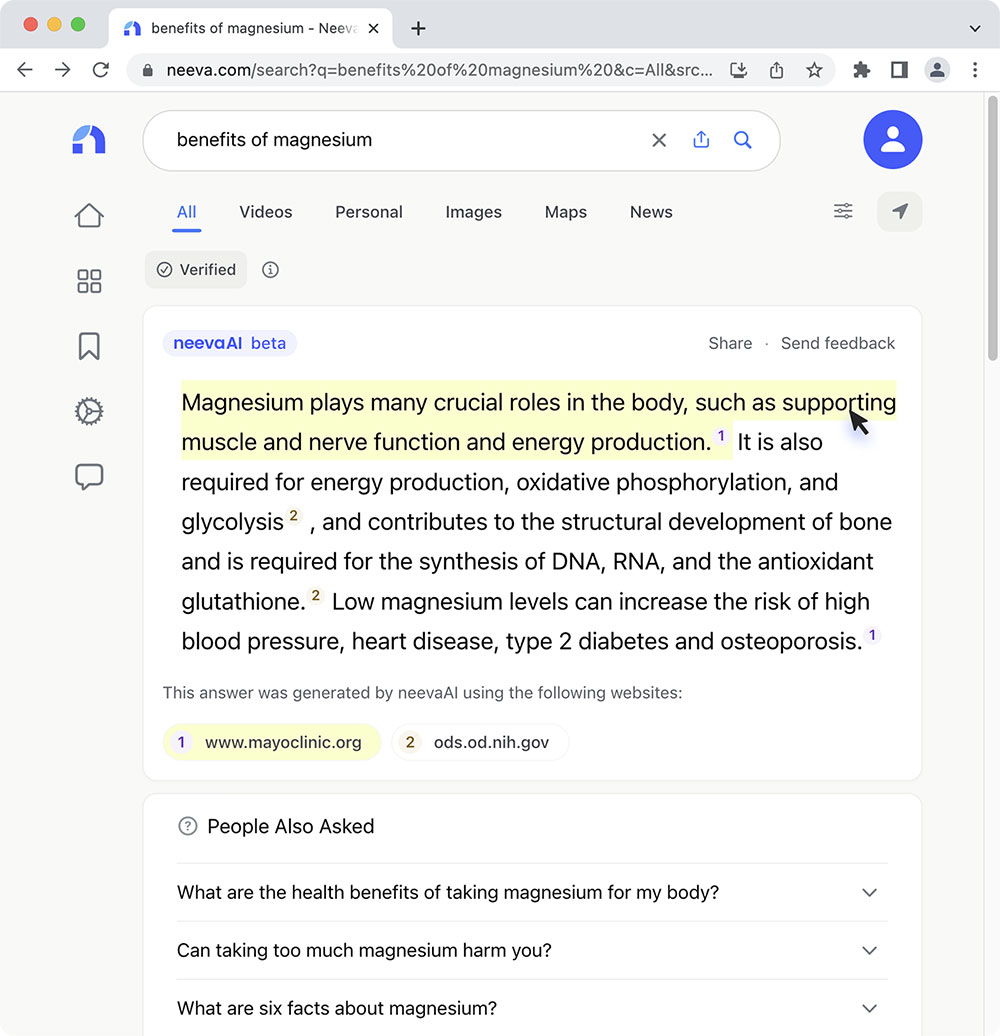This is a detailed descriptive caption for the given screen capture:

---

**Detailed Caption:**

The screen capture begins with a gray bar at the top featuring three colored circles—red, yellow, and green—followed by text reading "benefits of magnesium." Additionally, a blue "U" icon is visible, indicating the website, which appears to be Nivea.com. The browser toolbar includes a back arrow, forward arrow, refresh icon, and a padlock symbol in the search bar indicating a secure connection.

Further across the toolbar, there are a series of icons: a box icon, another box icon, a star, a puzzle piece, a piece of paper, and a gray circle with a person icon. Three gray dots appear adjacent to these icons.

The background of the page transitions to a tan color with a white search box below the toolbar. The search box contains the text "benefits of magnesium" along with an X icon, a box icon, and a magnifying glass. Underneath the search box, in blue, the word "All" is highlighted, which is followed by other categories in gray: Videos, Personal, Images, Maps, and News.

On the right-hand side of the image, there are several icons for navigation: a house, a four-square grid, a ribbon, a cogwheel, and a text bubble—all in red and gray.

Below this bar, there is a gray box with the text "Verified" accompanied by a checkmark and an eye icon. This is followed by a white section with the text "Nivea AI Beta" in blue and "share some feedback" in gray. In this white section, there is black text, part of which is highlighted in yellow. The highlighted section reads:

"Magnesium plays many crucial roles in the body such as supporting muscle nerve function and energy production."

Next to the word "supporting," there is a black arrow pointing right. The continuation of the black text reads:

"It is also required for energy production, oxidative phosphorylation, and glycolysis, and contributes to the structural development of bone. It is required for the synthesis of DNA, RNA, and the antioxidant glutathione. Low magnesium levels can increase the risk of high blood pressure, heart disease, type 2 diabetes, and osteoporosis."

At the bottom, a note states that the answer was generated by Nivea AI using sources such as MayoClinic.org and ODS.OD.NIH.gov. Following this, a "People Also Ask" section lists related queries: "What are the health benefits of taking magnesium for our body?", "Can taking too much magnesium harm you?", and "What are six facts about magnesium?"

---

**End of Caption.**